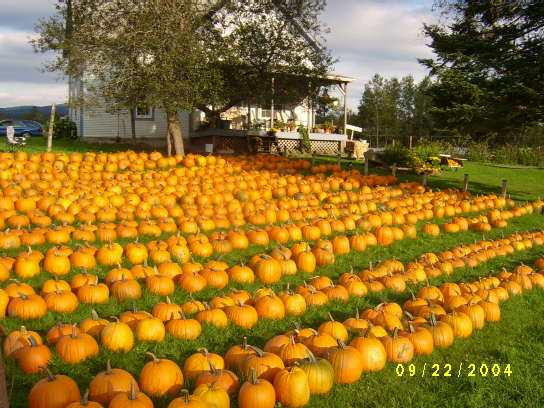The image captures a sprawling pumpkin patch set on a lush, deep green lawn, with numerous bright orange pumpkins meticulously arranged in rows that stretch from the bottom left to the top right of the frame. The rows, varying from two to three pumpkins wide, add a sense of abundance and meticulous arrangement typical of a fall harvest. Each pumpkin has a visible stem, indicating that they have been harvested and are ready for picking.

In the background stands a charming white, two-story A-frame house with a porch, likely part of a farm property. A shade tree with green leaves stands in front of the house, adding a touch of natural elegance. Behind the house lies a tree line, possibly indicating additional farmland or woods, and a distant mountain range adds a majestic backdrop to the scene. The sky above is predominantly cloudy with occasional patches of blue, suggesting a serene, late summer or early fall day. Additional details include a car and a chair on the lawn, garden beds with circular sections of flowers, and a date stamp at the bottom right corner reading 09-22-2004, grounding the scene in a specific moment of time.